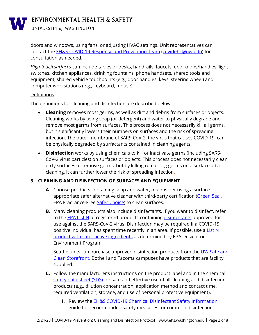This image primarily features a white background with black text, interspersed with blue hyperlinks. Dominating the visual field is a prominent "W" logo, accompanied by another emblem related to Environmental Health and Safety. The text is structured in bullet points, although the paragraphs themselves are largely illegible. The overall appearance is one of a document or webpage with standard formatting, where specific content remains unreadable except for a few recognizable elements.